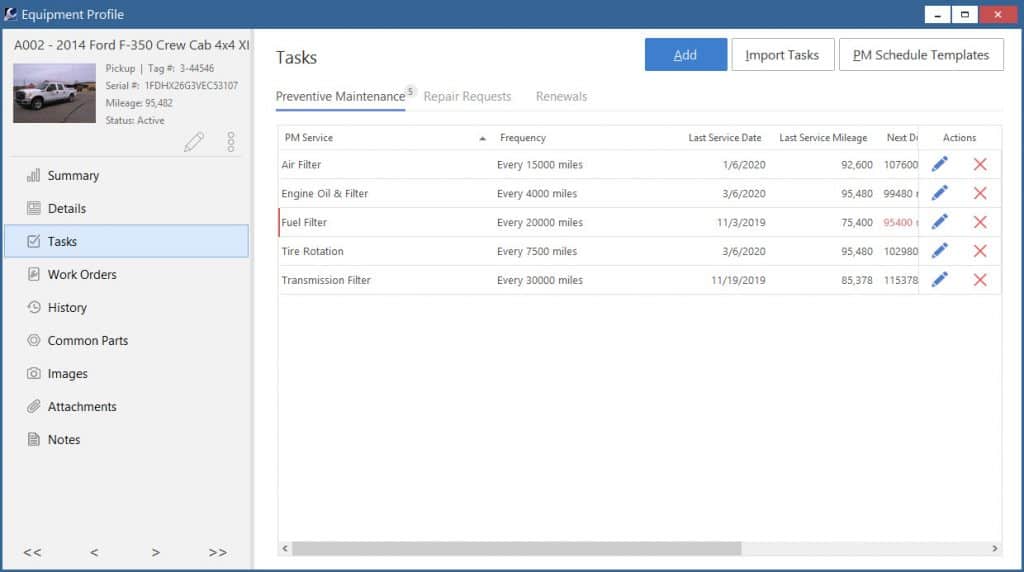The image is a screenshot from a website, showcasing a detailed equipment profile interface. The top bar is blue, displaying the title "Equipment Profile," with Expand, Minimize, and Close buttons situated in the upper right corner. On the left side, there is a vertical panel which includes information such as "A002-2014 Ford F350 Crew Cab 4x4 XL," accompanied by an image of the vehicle. Additional details in this section include the pickup's tag number, serial number, mileage, and its active status. Below this, several categories are listed: Summary, Details, Tasks, Work Orders, History, Common Parts, Images, Attachments, and Notes.

The right side, which occupies three-quarters of the screen, primarily displays the "Tasks" section. Within this section, there are tabs for Preventative Maintenance, Repair Requests, and Renewals. The Preventative Maintenance tab is currently highlighted, showing a list of items such as PM Service, Air Filter, Engine and Oil Filter, Fuel Filter, Tire Rotation, and Transmission Filter. Each item includes columns for Frequency, Last Service Date, Last Service Mileage, and Actions, with options to edit these entries. At the top of this section, users can select from three options: Add, Import Tasks, or PM Schedule Templates.